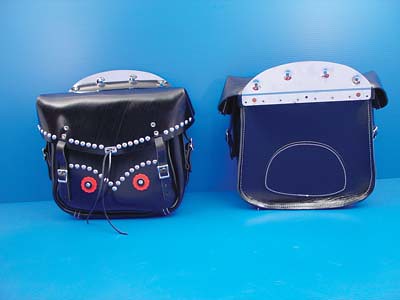This image is a highly detailed color photograph depicting motorcycle saddlebags against a vivid background. Both the wall and the surface on which the saddlebags rest are different shades of blue, creating a striking contrast. The left saddlebag showcases intricate details: it features a black leather cover that tapers to a slight point in the center, adorned with silver studs forming a decorative V-shape. Additionally, two red-blue leather accents embedded with silver brads give an impression reminiscent of eyes, adding character to the bag. The cover is secured by two leather straps with chrome buckles, giving it a rugged yet stylish look. The back of this saddlebag is plain blue with visible metal mounts designed to attach securely to a motorcycle. The right saddlebag appears more simplistic, dominated by a smooth blue leather surface. The interior flap is white and features small metallic knobs, enhancing its functional yet understated design. Overall, these bags are meticulously presented, leaning against a backdrop that accentuates their vibrant colors and detailed craftsmanship.